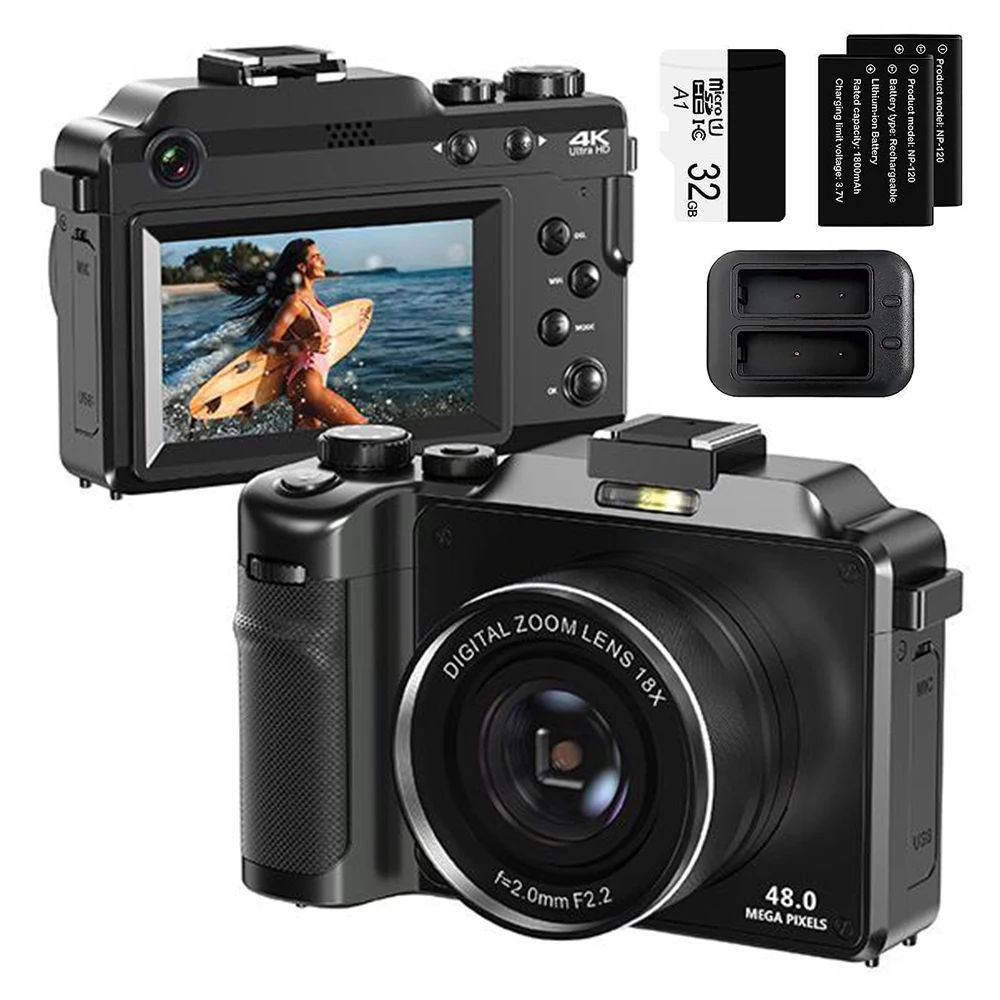This image is an advertisement for a digital camera, featuring a detailed display of the front and back views of the camera. The camera, which is entirely black with white text, prominently showcases a "Digital Zoom Lens 18x" and "48 megapixels" on the front. It also includes technical specifications such as "f = 2.0mm, f/2.2" beneath the lens. The front view highlights the main lens, while the back view displays an LCD screen showing an image of a tan woman in a pinkish bikini holding a beige surfboard and walking into the ocean. This screen is labeled with "4K HD," indicating high-definition video capabilities.

In addition to the camera views, the advertisement also features accessories included in the package. Positioned in the top right corner, there are images of micro SD memory cards, with one labeled as 32 gigabytes, two slim lithium batteries, and a battery charger. The overall composition effectively highlights the camera's features, accessories, and visual quality through the example image displayed on the LCD screen.